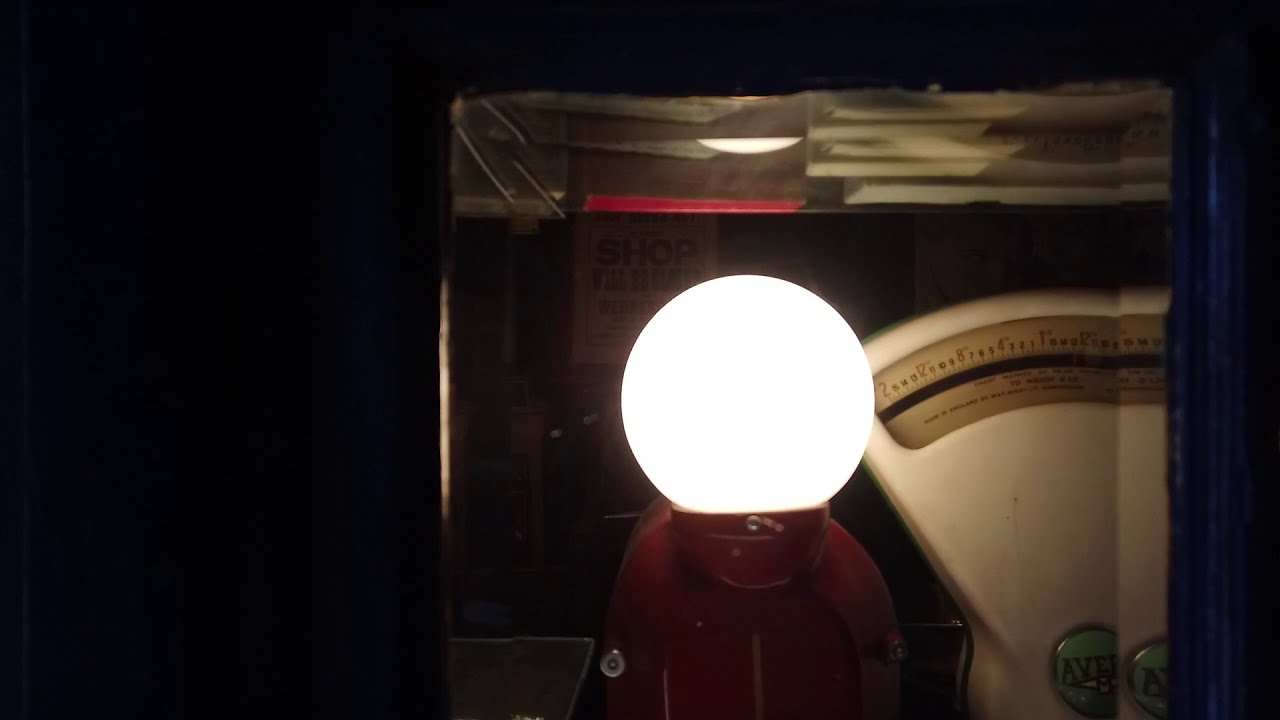The image depicts a dimly lit storage room or office dominated by a strikingly bright, round lamp that resembles a crystal ball. The lamp is perched on a red metal base, emitting an intense white light that creates a stark contrast against the otherwise dark surroundings. Adjacent to the lamp is a vintage butcher scale, characterized by its white, fan-shaped top and an arched bar with numbers. The scale features a green circle bearing the letters A-V-E-E. Behind these objects, a stack of plastic boxes filled with paperwork is visible, alongside a red binder. A mirror above the scene reflects the bright lamp and the top of the scale, enhancing the room's illumination. Additionally, an old-fashioned sign with the word "SHOP" is partially visible, further accentuating the room's nostalgic atmosphere.